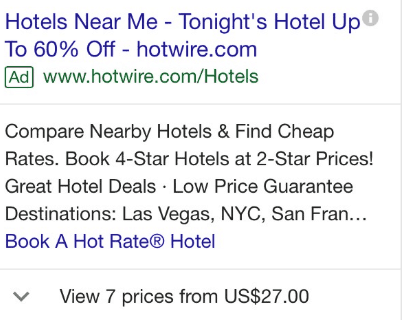This is a screen capture of a sidebar advertisement for Hotwire.com focused on hotel bookings. The ad prominently features a headline in blue text on a white background, which reads, "Hotels Near Me Tonight - Up to 60% Off | Hotwire.com." Beneath this, green text indicates the ad label and URL: "Ad www.hotwire.com/hotels." The ad encourages users to "Compare nearby hotels and find cheap rates. Book four-star hotels at two-star prices. Great hotel deals, low price guarantee." Destinations like Las Vegas, NYC, and San Francisco are mentioned, although the text is truncated with ellipses.

Another blue link, "Book a Hot Rate® hotel," is present, highlighting Hotwire's trademark offer. A dropdown menu displays, "View 7 prices from $27 USD." The ad is set against a white background with thin light-gray lines demarcating each section. The text is primarily in black, and a small gray icon featuring a white "i" suggests additional information can be accessed without leaving the search engine page. This ad is minimalistic and structured for quick, at-a-glance information consumption.